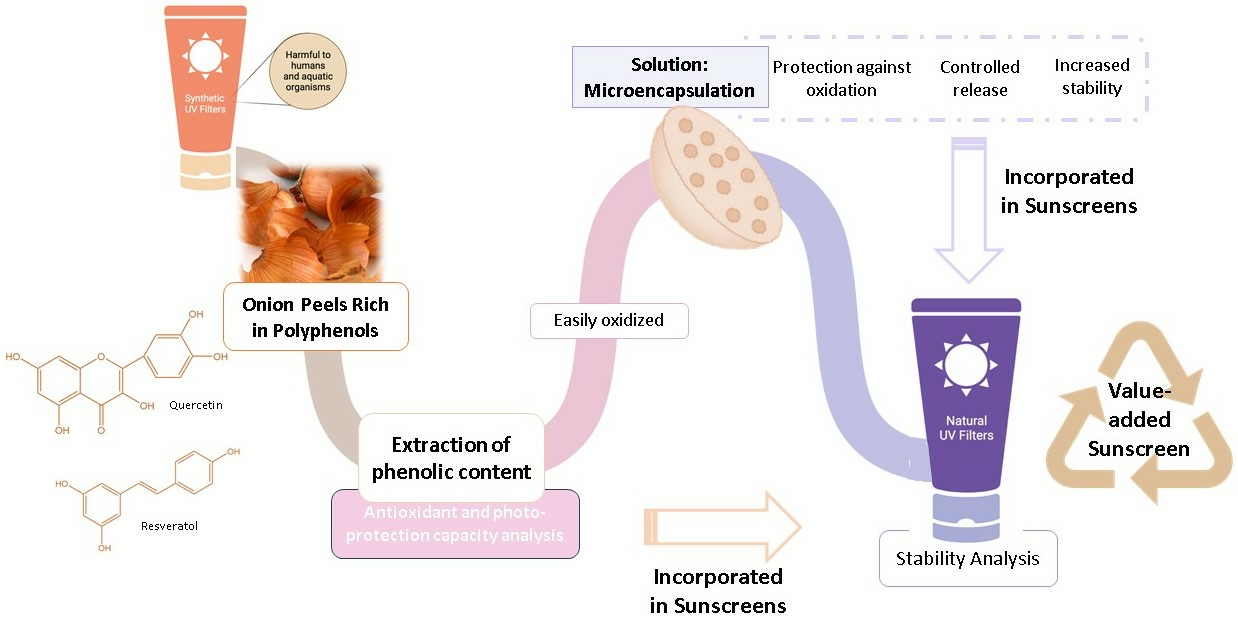The image is an informational diagram set against a white background, illustrating the components and processes involved in the creation of a specialized sunscreen. The rectangular diagram features multiple lines of black text and images, with the top and bottom sides being twice as long as the left and right sides. 

Starting from the left, a cartoon rendition of a tube of lotion, labeled "harmful to humans and aquatic organisms", showcases a front label reading "synthetic UV filters". Below this, an image of brown onion peels is highlighted with the text "onion peels rich in polyphenols". A line from this image leads to another text segment that outlines the "extraction of phenolic content, antioxidant and photo protection capacity analysis".

Further details in the diagram include a process description: "equally oxidized" substances undergo "solution, microencapsulation," which results in "protection against oxidation, controlled release, and increased stability". The diagram concludes with a note on its purpose, which is to highlight the benefits of these ingredients for a "value-added sunscreen". This detailed flow indicates not only the harmful impact of synthetic UV filters but also the beneficial inclusion of natural elements like onion peels in sunscreen formulations for enhanced effectiveness and stability.